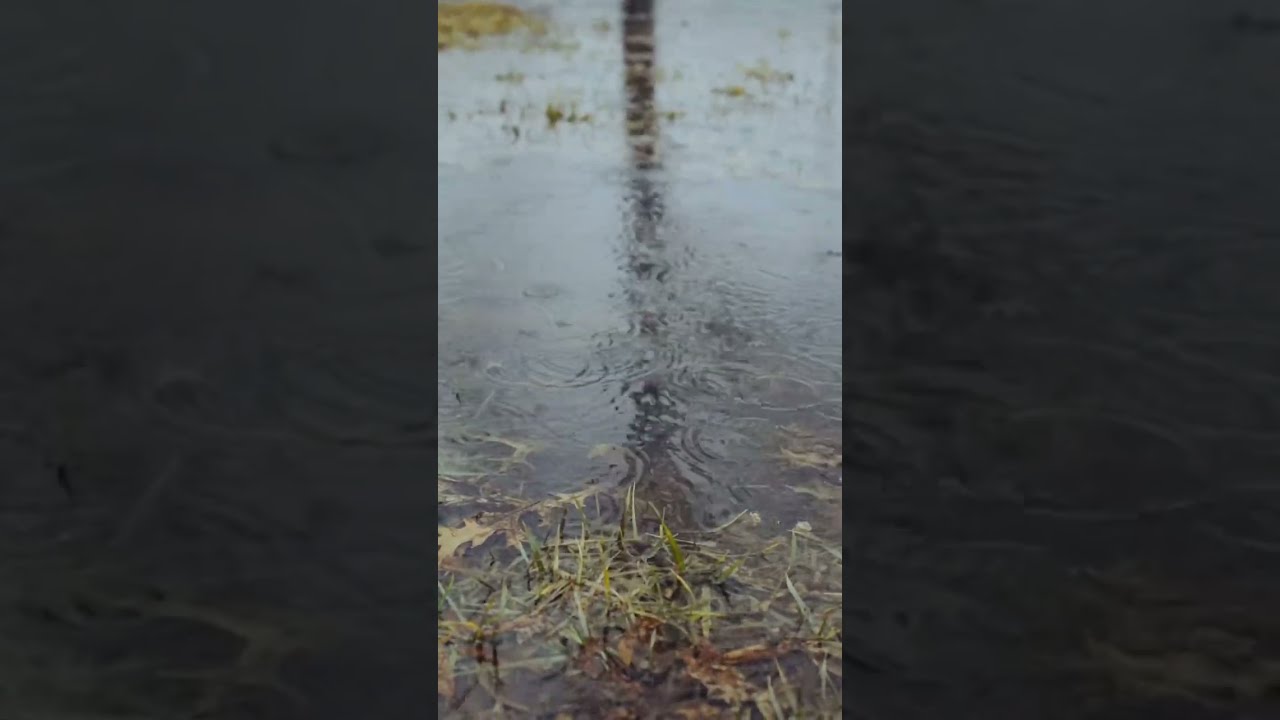This photograph depicts a small section of a murky pond or swamp, its greenish-gray water reflecting the shadow of a tree trunk from above. Visible on the water's surface are gentle ripples, suggesting either recent rain or a light breeze. In the foreground, clusters of green and brown leaves—possibly fallen or emerging as seasons change to spring—add a tactile depth to the scene. Amid these details, a submerged creature, likely an alligator, can be seen, with its head cloaked in loose grass and its tail trailing back into the water, blending seamlessly into the natural surroundings. The image, framed in a smartphone-like aspect ratio, appears slightly dark, indicative of an overcast or cloudy day. The photograph is bordered by dark, almost black sections, one of which contains a close-up of the water, giving the overall composition a segmented, cinematic feel.